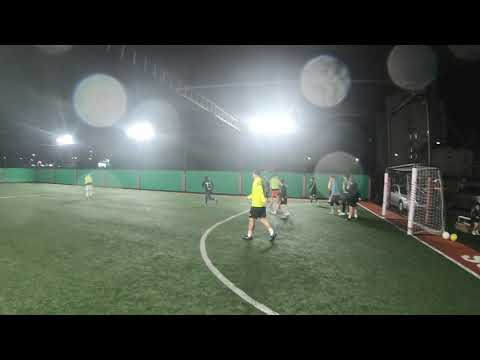The image depicts an outdoor nighttime soccer practice on a well-lit field under a black sky. Three powerful stadium lights illuminate the scene, with the closest light being central in the frame and two others receding towards the left. The players, dressed in exercise clothing rather than uniforms, occupy an artificial grass field marked with white lines delineating the goalie area. Most players are garbed in darker colors like black, dark blue, or gray, except for the closest player to the camera, who stands out in a bright yellow shirt and black shorts. A person on the left in the background can be seen running, dressed in black pants. The soccer goal is situated on the right-hand side, surrounded by several players, with a couple of spare soccer balls visible nearby. The field is encircled by a high green fence, and behind it, there is a strip of brown ground where a silver car and another vehicle are parked. The background reveals a faint outline of town buildings on the right side, accentuating the outdoor setting. The landscape-style image is framed with black bars on the top and bottom, suggesting an aspect ratio adjustment to fit the frame.